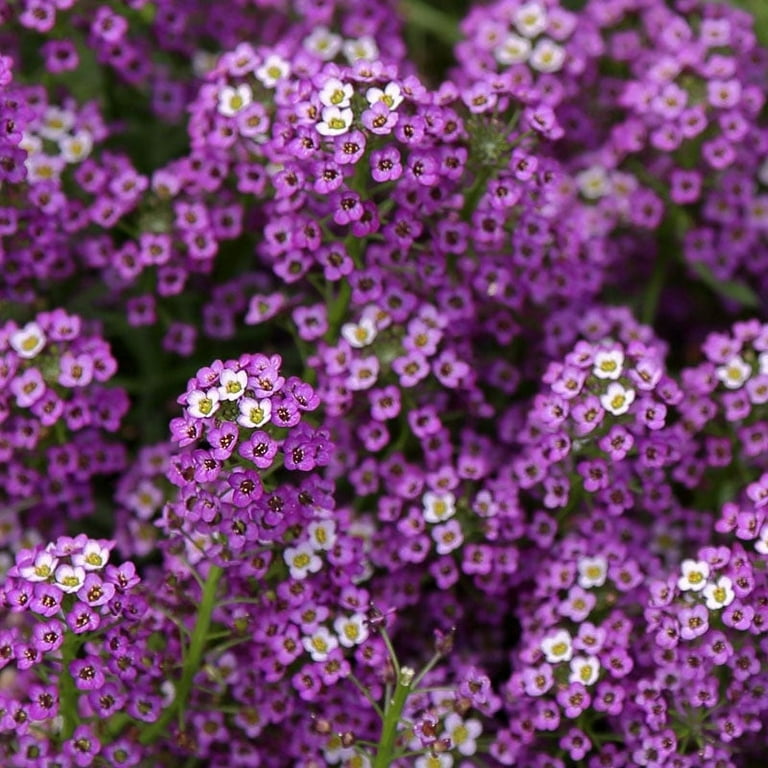This detailed photograph captures a professionally-shot image of numerous small flowers, predominantly purple and white, likely clustered outside a garden. The flowers, which might be violets, are accompanied by green stems and veins, with a few sprigs of green grass interspersed. The purple flowers come in various shades, mostly medium, and feature red centers with yellow tints, while the white flowers have lime green centers tinged with red. The flowers are arranged in dense clusters, with some in sharp focus and others blurred in the background, giving the picture a dynamic depth. The overall color palette of the image includes shades of purple, white, green, and hints of brown and black, with no other plants, animals, or activity present. The attention to detail and quality of focus suggests a professional level of photography.